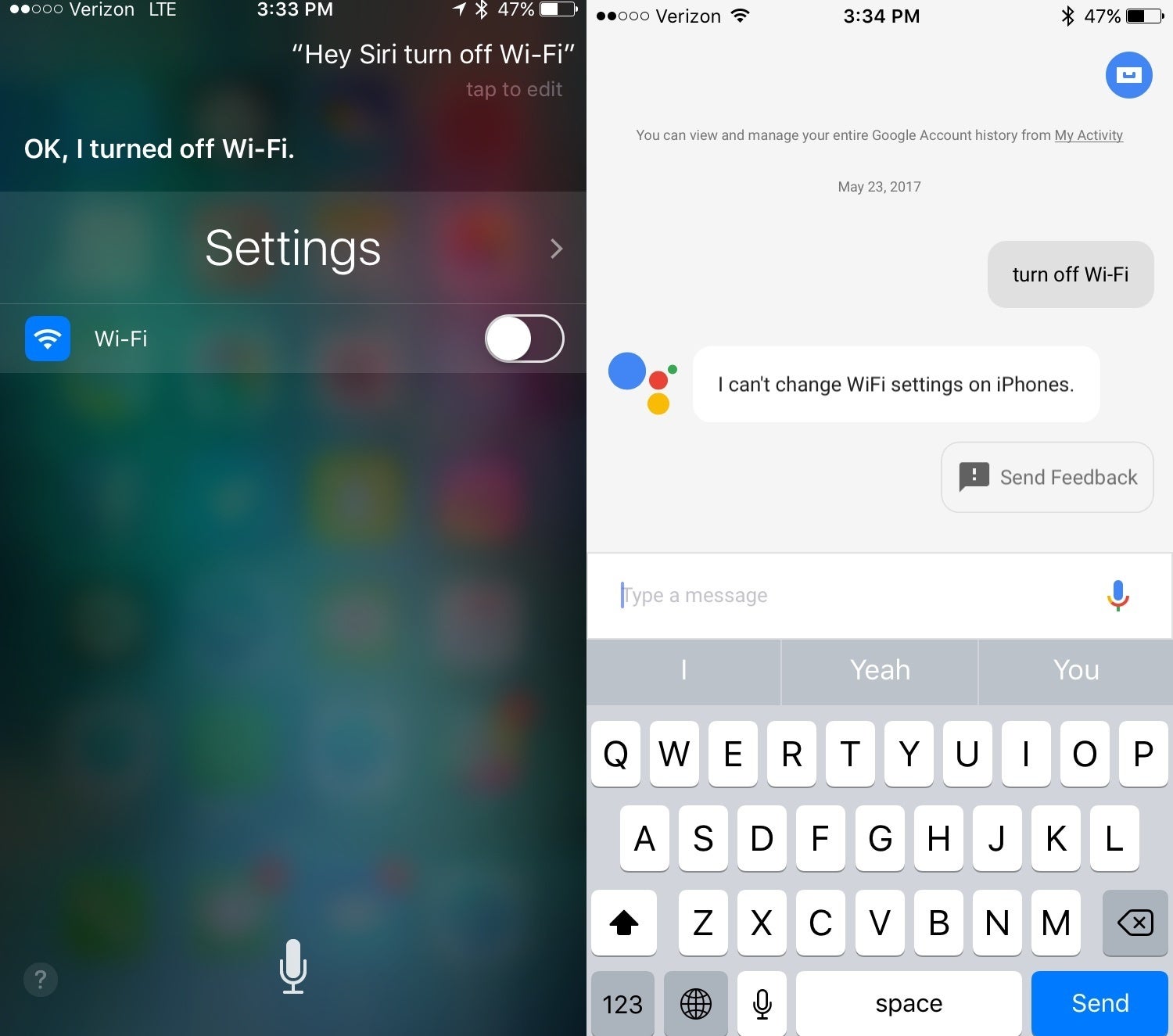The image is divided into two sections, each displaying a conversation with a virtual assistant.

**Left Side: Siri Conversation**
- **Header:** "Hey Siri, turn off Wi-Fi"
- **Siri’s Response:** "Okay, I turned off Wi-Fi."
- **Additional Info:** Visual confirmation shows the Wi-Fi settings screen where the Wi-Fi toggle switch is set to 'off.' The background is a blurred home screen with indistinct green, black, and various app colors.

**Right Side: Cookie Assistant Conversation**
- **Header:** "You can view and manage your entire account history from My Exhibit. May 23, 2017"
- **User Command:** "Turn off Wi-Fi" (Displayed in a gray text box with black text)
- **Cookie Assistant's Response:** "I can't change Wi-Fi settings on iPhones." (Displayed in a white text box with black text and an icon of four circles in blue, red, yellow, and green to represent the Cookie Assistant)
- **Footer:** Option to "Send Feedback," accompanied by a white keyboard and a blue 'Send' button at the bottom right.

**Background Information for Both Sections:**
- The Cookie Assistant conversation is set against a gray background, whereas Siri’s interaction has the home screen of the device blurred in the backdrop, showcasing green, black, and various other colors of the apps.